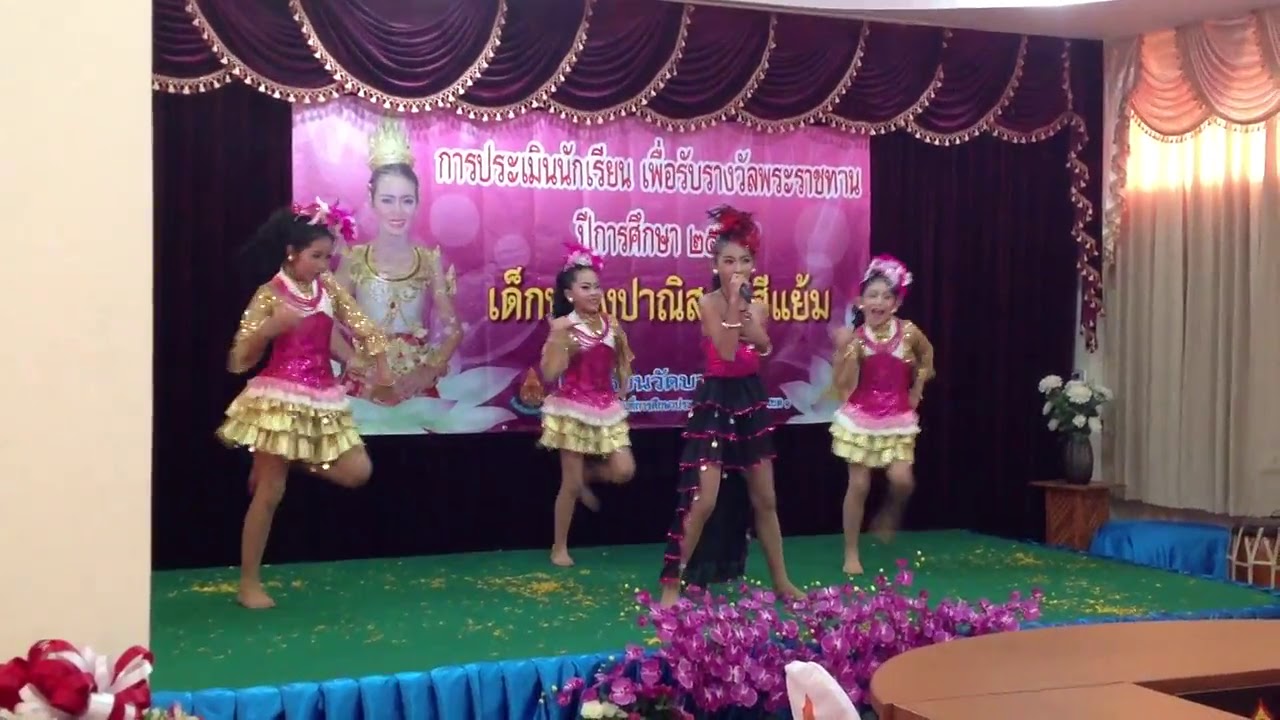In the image, four young girls, around age 10, are performing on a green stage with blue and purple curtains and a backdrop featuring a large pink sign with a woman and non-English text, likely from a South Asian language. The stage surface appears to be textured, resembling green astro turf. The performance is led by a girl at the front, dressed distinctively in a short black dress with a longer back, adorned with pink frills and a pink tank top underneath. She holds a microphone in her left hand, singing, with red feathered decorations in her hair.

Behind her, three backup dancers stand in a line, tallest to shortest from left to right. They wear matching gold skirts and pink tops with gold frills on the arms. Each girl has black hair styled in ponytails, accented with pink flowers. All the dancers are in a synchronized pose, raising their right legs. At the bottom of the photo, purple flowers are visible, suggesting a decorative element for the competition or event where they are performing.